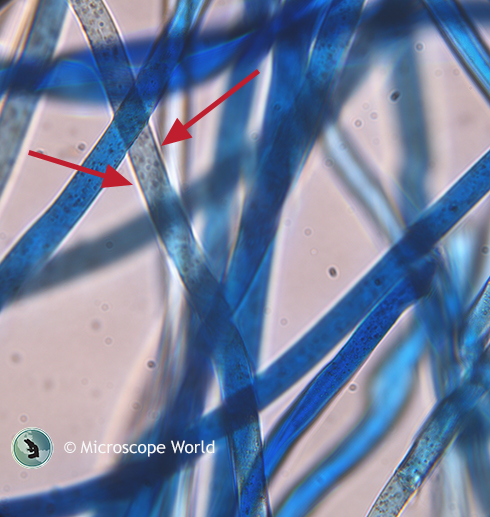This detailed photograph, titled "Microscope World," captures a complex microscopic scene on a white background. The image predominantly features long, blue translucent ribbons crossing in various intricate patterns, resembling strands of some material. Within these ribbons are small dark flecks or dots, indicating possible microscopic details or particles. 

Two red arrows are prominently placed, directing attention to one specific ribbon that stands out due to its lighter, almost white appearance, contrasted with black spots inside. This particular strand is less blue than the others, suggesting a point of interest or anomaly that the observers want to highlight.

Interspersed throughout the scene are various speckles and pieces of debris, adding to the complexity of the image. At the bottom of the photograph, there's a circle containing an indistinct, greenish figure, possibly an organism like a frog or amoeba. This element, along with the red arrows, emphasizes the scientific and exploratory nature of the image, underscored by a "Microscope World" label and copyright notation. The overall composition suggests a meticulously captured microscopic world, inviting viewers to examine its detailed and layered structures closely.